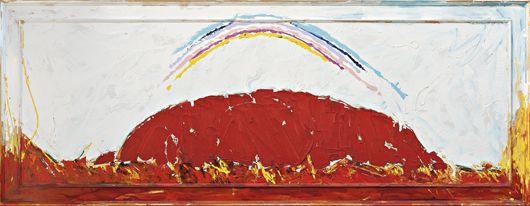The image depicts a horizontally oriented, long rectangular painting with a predominantly white background peppered with hints of turquoise, especially noticeable in the top right corner. The central focus of the artwork is a large, irregularly shaped red lump, reminiscent of Ayers Rock. This red form dominates the middle of the canvas, positioned on a ground that transitions from red to yellow hues, with gold lines providing highlights and additional texture.

Above this red mass, a rainbow arches across the canvas, displaying a spectrum of colors including light and dark blue, pink, and yellow. The strokes of the rainbow are primitive and rough, with the colors blending in a somewhat haphazard manner, giving the work an unrefined, raw aesthetic. The rainbow's vivid colors contrast sharply against the backdrop, further emphasizing its presence.

The bottom part of the painting mirrors the color palette seen in the ground beneath the red form, with shades of red, yellow, and orange blending together. Overall, the painting exudes a sense of raw energy and abstract composition with bold, unrestrained brushstrokes.